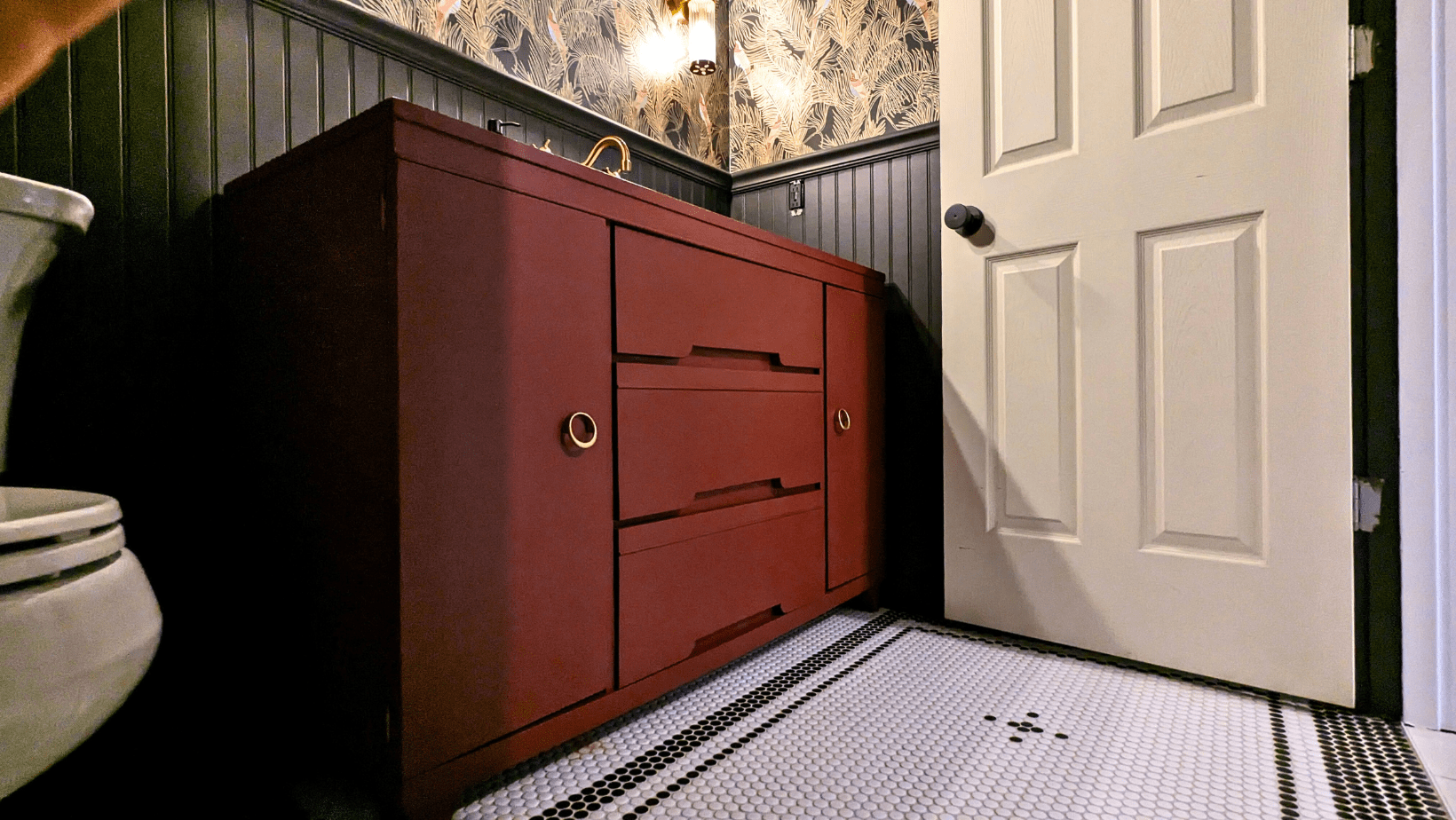The photograph captures an elegantly decorated and meticulously maintained bathroom viewed from a low angle in a corner. To the far left, a white toilet is partially visible. The lower half of the walls is adorned with hunter green wainscoting, while the upper half showcases intricate wallpaper with a green leaf pattern against a beige background. The central focus is a modern, sleek vanity made from cherry wood, featuring two doors on the sides, three middle drawers, and gold hardware. Atop the vanity is a gold faucet, with only the water spout visible from the camera angle, and a soap dispenser. The floor is covered with small white octagon tiles, bordered by tiny black tiles. A unique design made with approximately six or seven black tiles forms a plus sign in the center. An open cream-colored colonial door with a black handle leads into this well-appointed space.